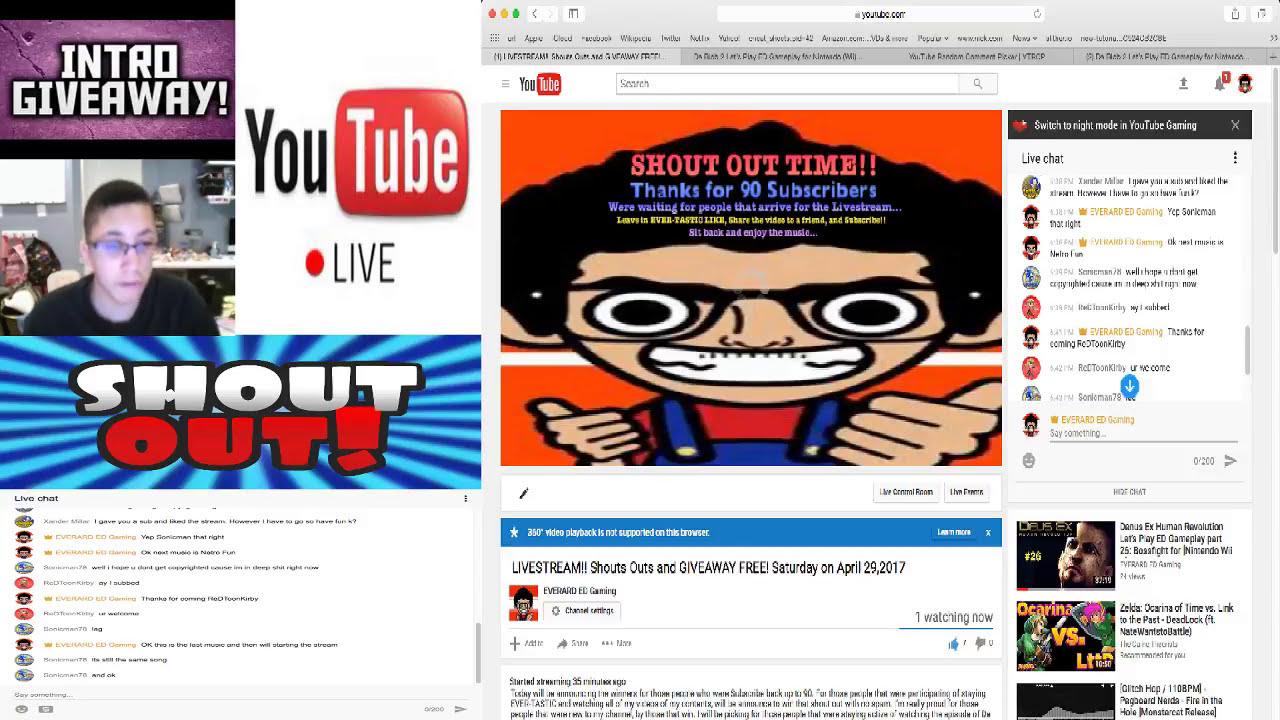The image displays a detailed screenshot of a computer screen showcasing a YouTube page alongside a pop-out window from another YouTube page. On the left panel, there is a thumbnail titled "Intro Giveaway, YouTube Live Shout Out" set against a purple background with white text. This panel features a young man with very short black hair and glasses, looking sideways. The section also has various smaller writings and icons beneath the thumbnail and shows live chat comments underneath in a continuous feed.

On the main right side of the screen, the YouTube interface is visible. In the center of this section, an illustration features an anime-style character with black hair, glasses, and a broad toothy smile, giving two thumbs up. The character is dressed in a blue jumpsuit and red shirt. Above the video is the usual YouTube header with the search bar, and a red "live" dot indicating that the streaming is happening in real-time. The video is titled "Shout Out Time, Thanks for 90 subscribers," with text and channel information found just below. Surrounding this are the typical elements of YouTube, including live chat on the right with numerous user comments, and suggestions for related videos and channels at the bottom right. The overall design highlights a celebratory shout-out related to a giveaway event, engaging live chat, and various interactive elements common to live streams on YouTube.